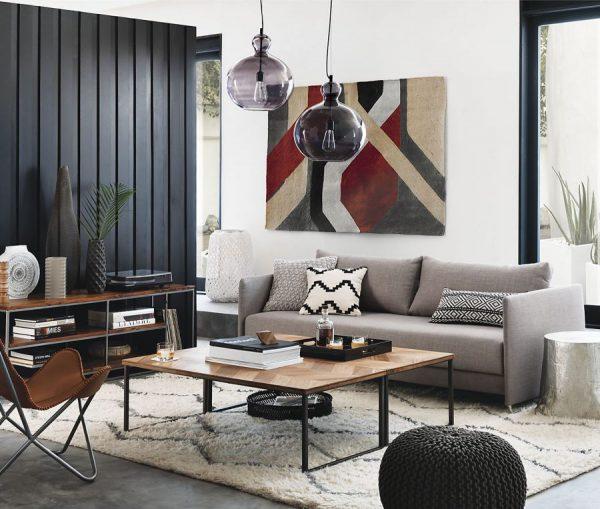This photo showcases a contemporary living room designed with a modern aesthetic in a smaller space. The room features contrasting walls, with one side covered in black wood shiplap, and the other painted white, with black trim accentuating the structure. A sleek gray tweed sofa against the back wall is adorned with a variety of pillows in shades of gray, white, and black. Above the sofa hangs a large canvas portrait composed of geometrical shapes in black, red, tan, and white.

The floor is covered by a large tan rug with black geometric lines that add a dynamic visual element to the room. Positioned on the rug is a brown wooden coffee table with black metal legs, which hosts a collection of books, a black round tray with candles, and another black tray underneath.

On the left side, a half-size bookshelf or media center in wood is placed in front of the black wall, displaying a mix of books, vases, and a black vase with a plant. Additionally, a silver round end table stands next to a black pouf ottoman and a brown folding chair, providing extra seating and storage options. The room's contemporary yet cozy atmosphere is highlighted by the meticulous balance of dark and light elements, as well as the thoughtful arrangement of functional furniture and decorative pieces.